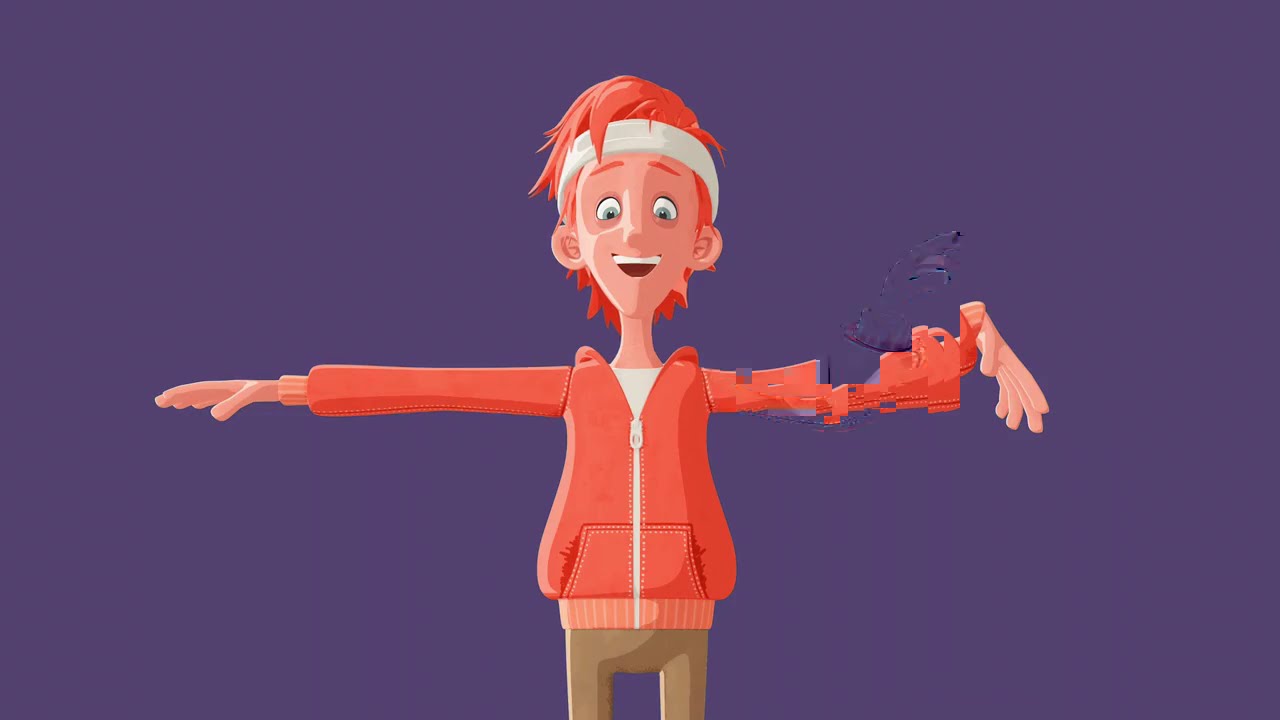The image depicts a slender, cartoon-like, 3D-rendered male character standing in the center of a solid dark purple background. The character has striking red hair and is adorned with a white sweatband around his forehead. His expressive face, with wide eyes and an open mouth suggesting surprise, adds a dynamic element to the scene. He is dressed in a vibrant orange hooded sweatshirt, which features a white zipper running three-quarters down its length, revealing a white shirt underneath. His attire is completed with olive or tan-colored khakis. The character’s arms are extended out to his sides, parallel to the ground. However, while his right arm and hand appear normal, his left arm is fragmented and distorted, exhibiting a glitchy, pixelated effect as though it is dissolving or malfunctioning.